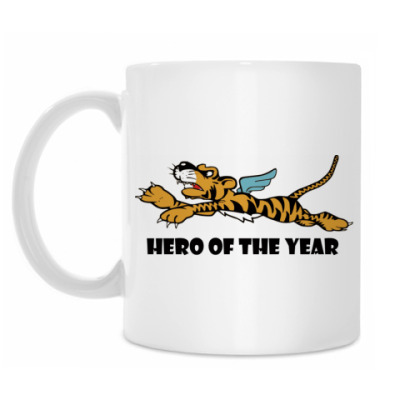This is a product image of a smooth, white ceramic coffee mug with a large handle on the left side. The mug prominently features a horizontal cartoon illustration of an orange and black striped tiger with blue wings, giving it a whimsical, flying appearance. The tiger, depicted with an assertive expression and claws extended, is positioned centrally on the mug. Below this illustration, the horizontal black text reads "Hero of the Year." The background of the image is pure white, emphasizing the mug's design and making it the focal point of the photograph.